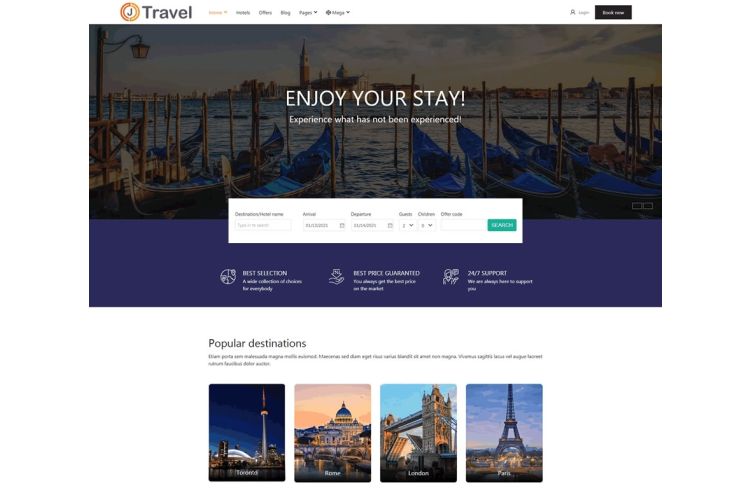This image is a detailed screenshot of a travel website designed to facilitate reservations. At the top of the website, there's a distinctive logo consisting of the letter “J” encircled, set against a gradient backdrop ranging from yellowish to brown hues. The site prominently features the word "Travel" in large, bold letters accompanied by several headings, including "Offers" and "Pages," though some are too small to read clearly. 

Located in the upper right corner is a login option next to a black clickable element. The background is adorned with a serene, slightly faded image depicting docked gondolas against the enchanting backdrop of Venice, with a view of St. Mark's Square and the cityscape extending across the beautiful, blue Venetian waters. Blue skies enhance the overall tranquility of the scene, which has been artistically tinted in deep blue tones.

The main interface includes various white text boxes inviting users to input their travel details such as destination, arrival date, departure date, number of guests, and children. A green "Search" button is positioned for easy access to initiate the booking process. Below these input fields, the site assures users with messages like "Best Selection," "Best Price Guaranteed," and "24/7 Support." 

Further down, the design showcases four thumbnail images of popular destinations: Toronto, Rome, London, and Paris, encouraging users to explore widely sought-after travel spots.